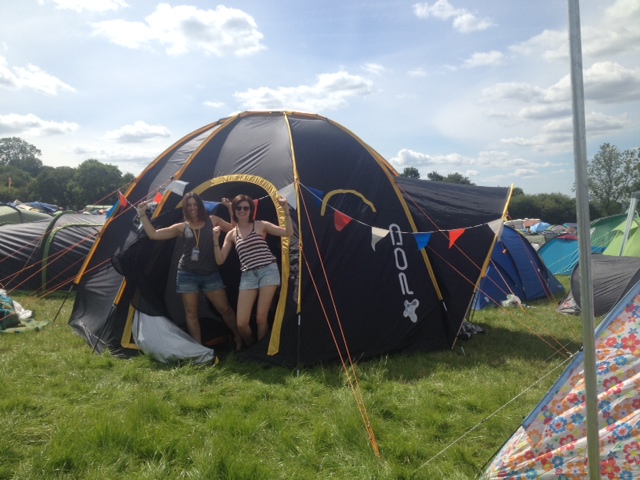The image depicts a vibrant scene reminiscent of a Woodstock-style party set within a lush, expansive grassy field. Dominating the foreground is an igloo-shaped, dark blue two-man tent adorned with yellow around the doorway, which is unzipped, revealing two Caucasian women with dark hair standing in its entrance. The woman on the left wears sunglasses, contrasts a red and white tank top, and blue cut-off shorts. The woman next to her is in a similar attire with a tank top, blue jean cut-off shorts, and dons a lanyard with a badge. They both stand energetically with their arms raised, adding to the lively atmosphere.

Scattered throughout the scene are various tents in an array of colors, including a tent with a floral pattern of orange, pink, and blue flowers on a white background with a blue outline, a green tent, and a dark blue one among many others. A notable silver tent pole stands prominently on the right side of the scene. Behind the mass of tents, lush trees with green foliage and brown trunks create a natural backdrop under a bright blue sky dotted with white clouds. The main tent in the center bears the label 'Pod' along with a pod symbol, presenting a mix of black and yellow on its exterior. Overall, the image captures a festive and dynamic camping event filled with nature and human exuberance.